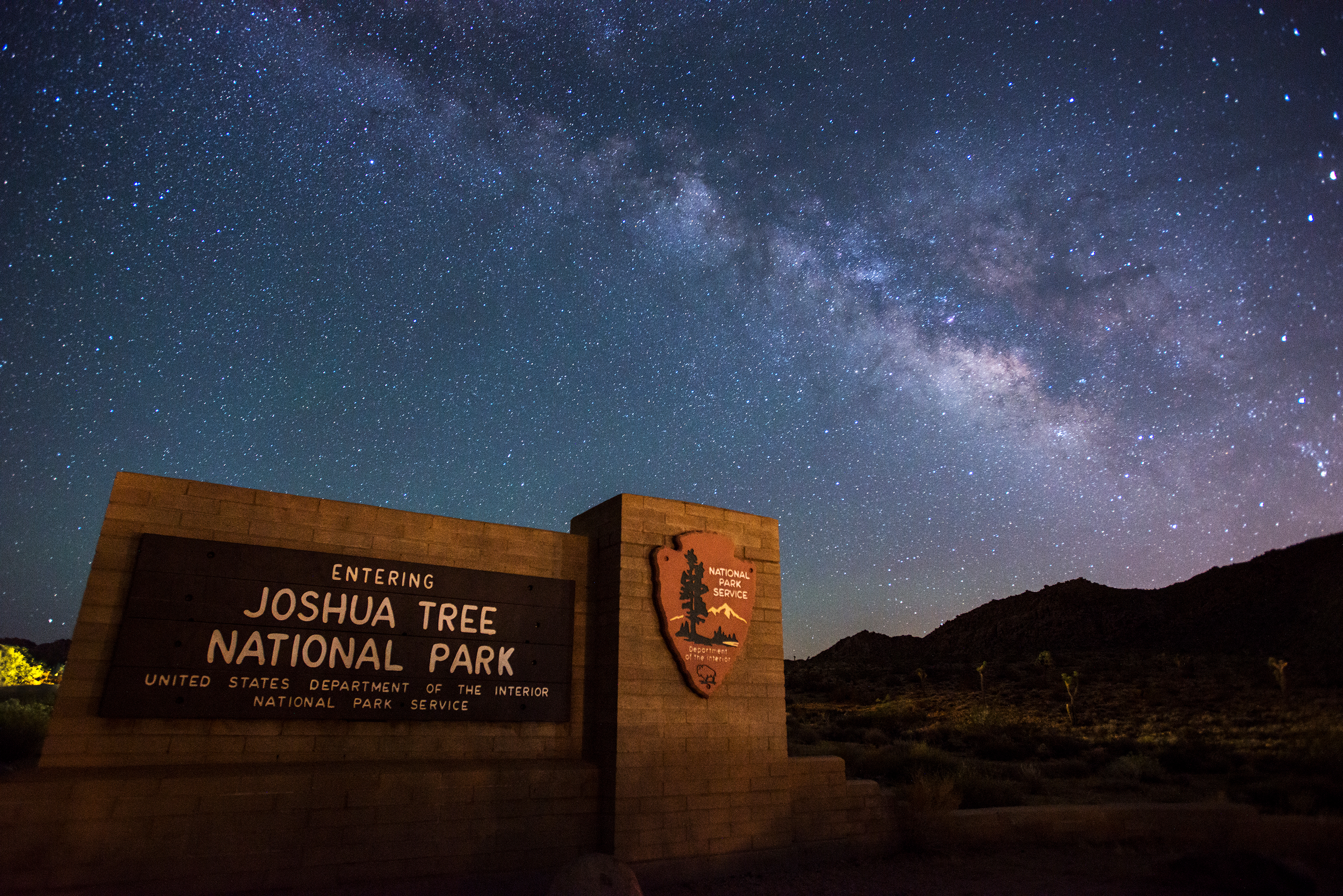The nighttime photograph captures the entrance sign to Joshua Tree National Park, prominently situated in the lower-left corner. The sign is an impressive brick and stone monument with an engraved plaque that reads, "ENTERING Joshua Tree National Park, United States Department of the Interior National Park Service." To the right side of the sign, there's a categorized plaque with additional writing and a picture. The scene, imbued with dark navy blue and tan hues, is framed by a vast, star-filled sky hinting at a setting moon. Subtle shadows reveal the silhouettes of hills and small trees in the background, painted by the remnants of twilight as the day transitions into night.